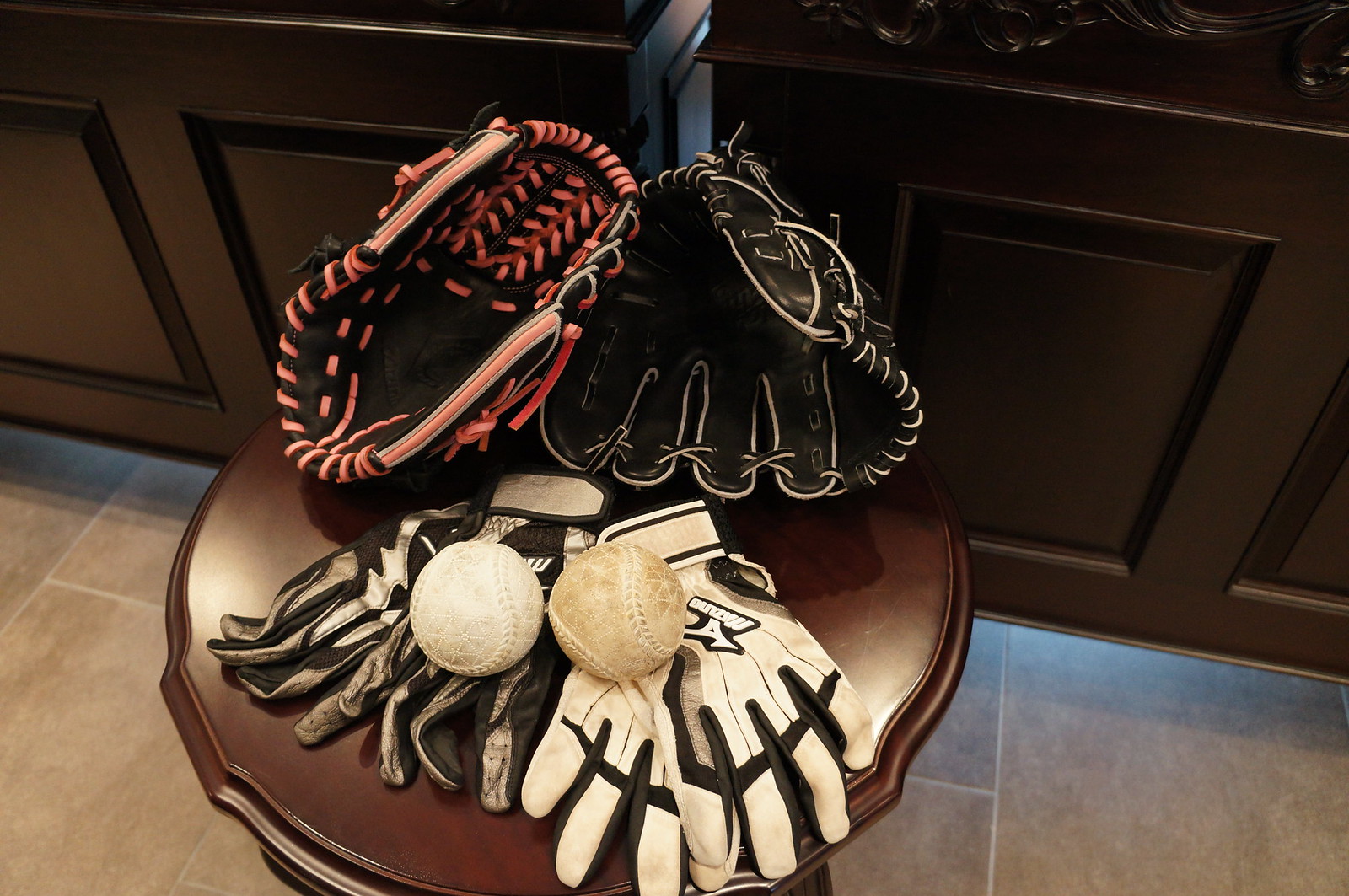This detailed color photograph captures an indoor scene featuring an assortment of baseball equipment meticulously arranged on a small, round, dark wooden table with slightly scalloped edges. The table is set against the backdrop of dark brown wooden cabinets, which may belong to a kitchen or office space, characterized by a dimly lit toe kick area. 

On the table, two distinct baseball gloves are prominently displayed: one is black with white stitching, and another is black with orange or pink threading. Accompanying these gloves are three pairs of black and white batting gloves, possibly Mizuno brand, varying in cleanliness with some appearing lightly soiled. Resting atop the batting gloves are two baseballs, one pristine white and the other bearing the marks of use, displaying a dirty brown hue. 

The room's floor is covered in grayish-brown stone tiles arranged with white grout lines, adding a subtle contrast to the warm tones of the wooden furniture and cabinetry. This image proficiently blends the rustic charm of wooden elements with the practical utility of sports equipment.